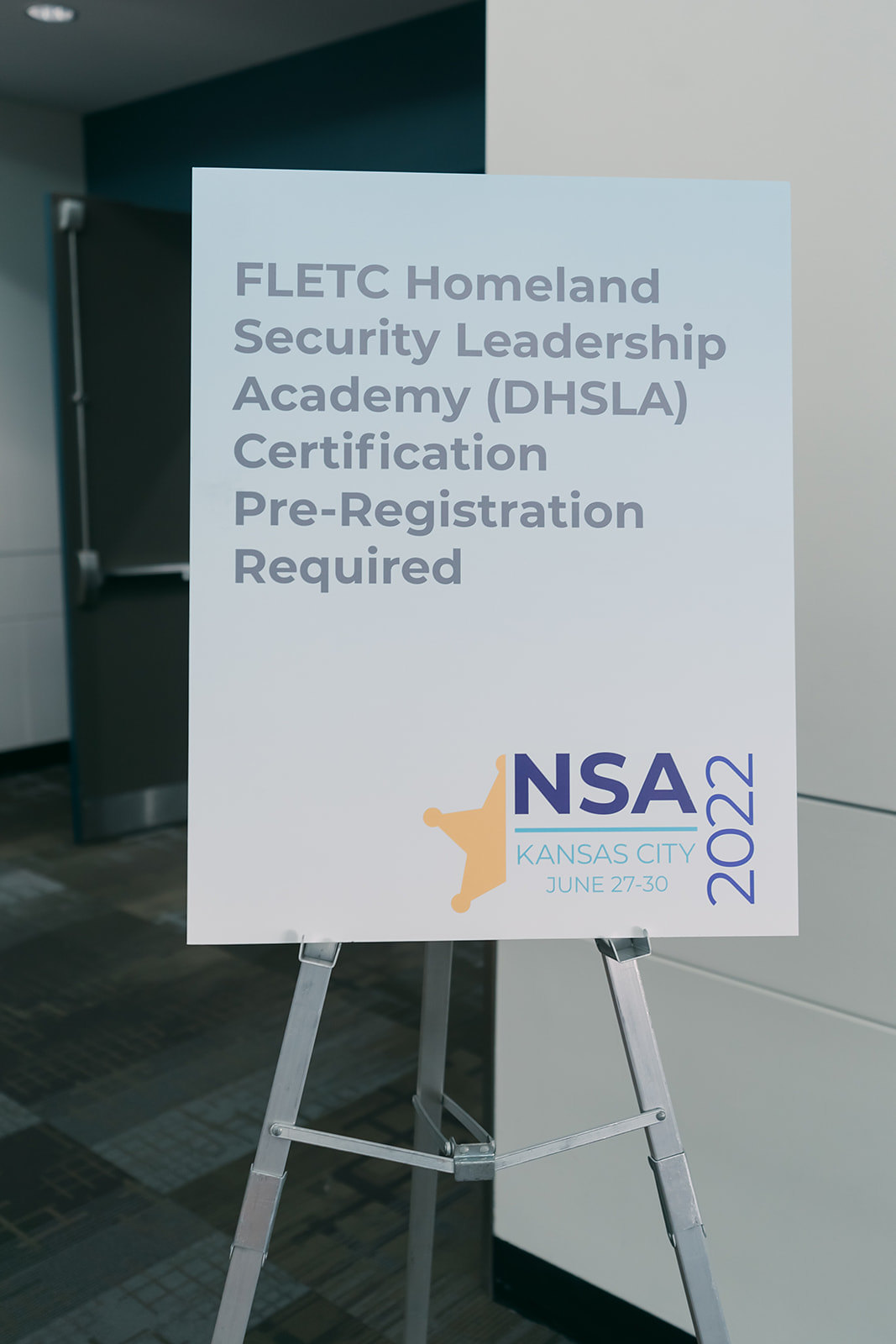This image features a detailed sign placed on a silver metal tripod stand, situated inside a professional business building. The tripod is positioned on square-patterned carpet, characterized by its black, gray, and white hues. The walls on the right side are white, while a set of industrial-sized double doors on the left side adds a utilitarian touch to the setting. A beige-colored wall and a dark hallway featuring a propped open dark-colored door are visible in the background.

The sign itself is a large rectangle with a gradient background shifting from light blue to white. The text on the sign, in various shades of gray and blue, reads as follows:

- At the top, in gray text: "FLETC Homeland Security Leadership Academy (DHSLA)"
- Below that, it states: "Certification Pre-Registration Required"
- In the bottom right corner, in large blue text: "NSA", with "2022" in light blue positioned vertically beside it
- Adjacent to the NSA text, part of a yellow sheriff's star is visible.
- Below NSA, it reads "Kansas City, June 27-30" in light blue text

The detailed layout and the careful placement of the sign indicate that it is for an important event, possibly a conference or seminar related to Homeland Security Leadership.